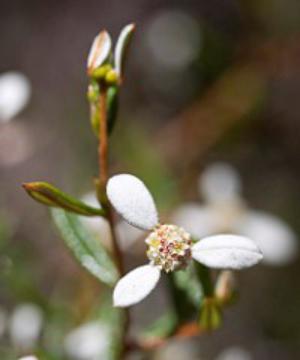This small, blurry image depicts flower buds that have not yet fully bloomed. The focal point is a partially opened bud, featuring three sparse, white petals extending from a colorful center with tiny dots in hues of yellow, red, and white. The surroundings include a mixture of green and brown stems and leaves, though the background is mostly indistinct due to a bokeh effect, with hints of additional plants and possible trees. There is also a second bud visible, less developed than the first, with closed green petals pointing upwards. The overall scene appears muted, with colors of brown, green, black, and white dominating a rather rough and unimpressive floral setting. Transparent white circles can be seen in the blurred background, adding to the image's low-resolution and unclear quality.